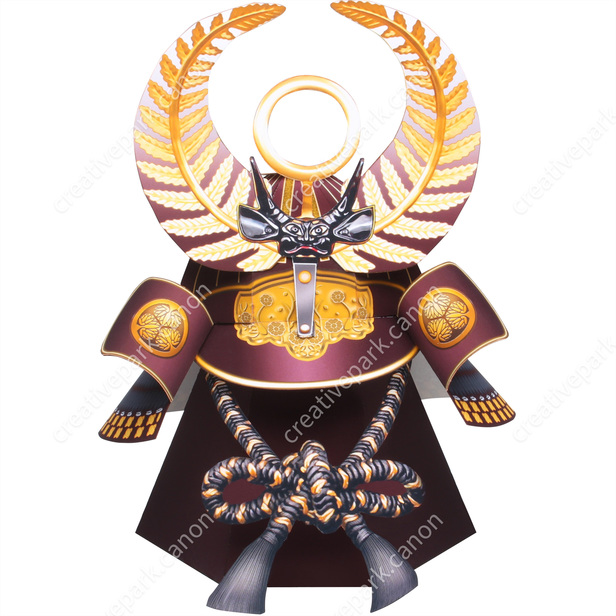This is a detailed color illustration of a traditional Japanese samurai helmet, facing the viewer, captured in a portrait orientation. The helmet features an ornate design with two curled sections on the forehead, each adorned with two gold circles and various gold squares along the outer edges. The dome of the helmet is purple, accentuated with gold stripes on the top, and capped with a gold rectangular crest adorned with intricate flower designs. 

A standout feature of this helmet is the silver clip, holding a stylized demon head with large pointed ears, eyes, and prominent horns. Extending from behind the demon head are two decorative elements that curl like horns, painted purple with gold leaf designs, enhancing the helmet's intricate appearance. Topping off the helmet, there's a golden circle at the very tip.

Additional details include tall, curved decorations resembling feathers or leaves that almost touch, painted in gold, and a central golden ring. Below the crest, there is a maroon and yellow cord bow with fringe at the bottom, attached to a black segment that resembles a skirt. The helmet's shoulders are accented with gold circular motifs and gold squares along the cuffs.

Overall, the illustration not only highlights the rich colors and detailed craftsmanship of the helmet but also includes a subtle watermark reading "Creative Park dot canon," indicating its digital origin from Creative Park by Canon.